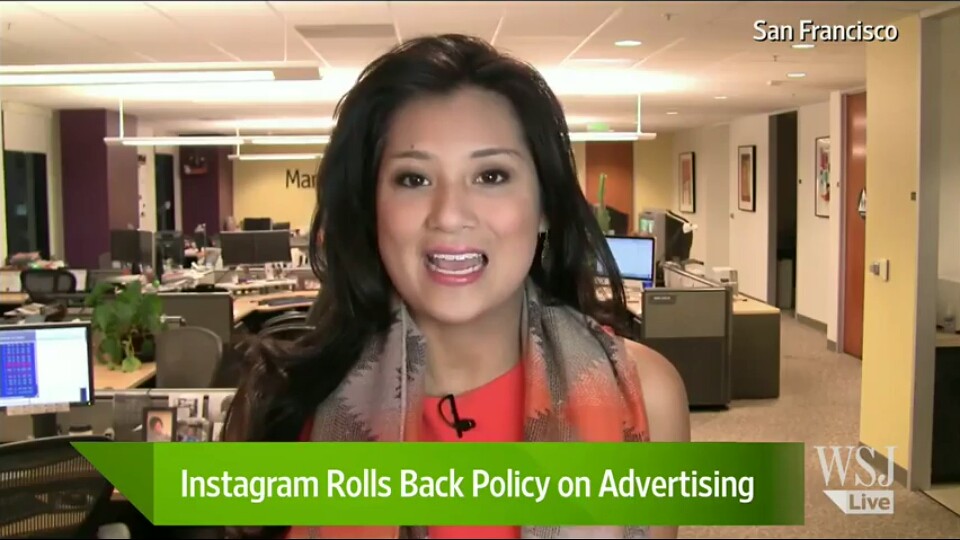This image depicts a young woman, possibly Latina, standing in an expansive office space that resembles a newsroom, filled with desks and computer monitors. The backdrop showcases the busy environment behind her, indicating she is on location. She has long dark hair and is wearing an orange shirt with a printed scarf over it. A small microphone is clipped to her shirt, suggesting she is speaking or reporting. In the lower left corner of the image, the white text reads "WSJ" and "live," identifying the broadcast as a live segment from the Wall Street Journal. The upper right corner of the image displays "San Francisco" in white text. A green banner at the bottom of the image conveys the news headline: "Instagram rolls back policy on advertising".